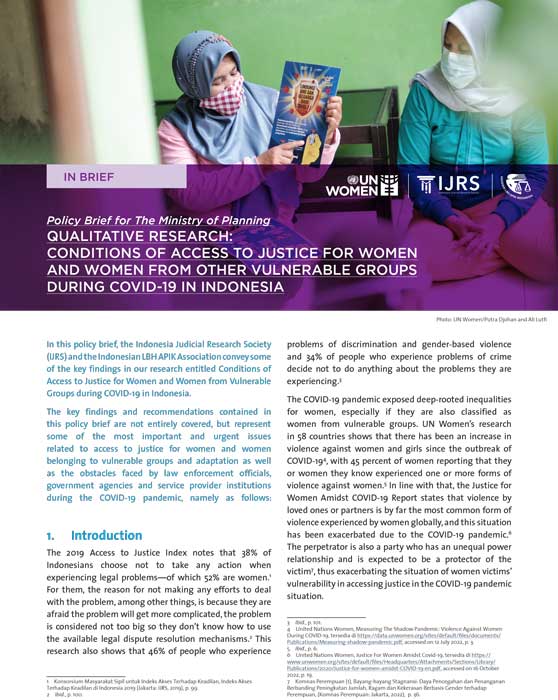The image features two women wearing hijabs, with their faces covered except for their eyes, suggesting they might be Muslim. The woman on the left is holding up a brochure, which the woman on the right is attentively looking at. The brochure seems to be an official document. Beneath the photo, in a purple section, there is text that reads: "Policy Brief for the Ministry of Planning: Qualitative Research on Conditions of Access to Justice for Women and Women from Other Vulnerable Groups During COVID-19 in Indonesia." This indicates that the context is related to the challenges faced by Indonesian women and vulnerable groups during the COVID-19 pandemic. Underneath the image, there are several small, light blue paragraphs that begin with "Introduction," suggesting a detailed explanation of the hardships experienced by these women during the pandemic.